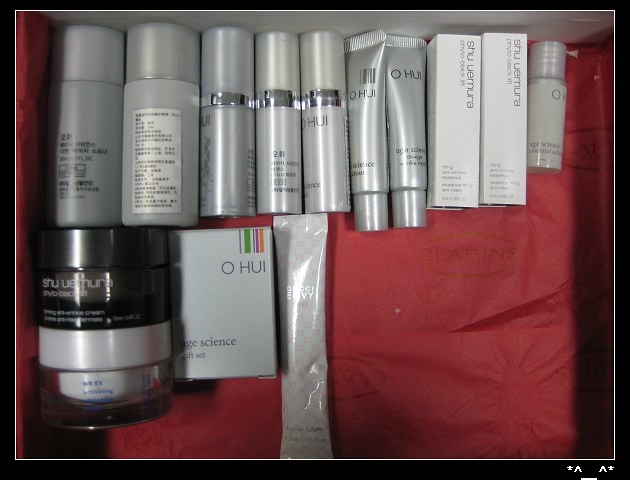The image depicts an open box lined with vibrant red paper, containing a selection of premium beauty products. Inside the box, there are several tubes and jars, each encased in sleek and shiny silvery-gray plastic packaging. The meticulous arrangement highlights the luxurious nature of the items. Prominently displayed among the products, the brand name OHUI (incorrectly identified as OHEAL) is written in clear text, suggesting high-quality skincare or cosmetic items. Additionally, the box includes products from another prestigious brand, Shu Uemura, often associated with top-tier beauty standards. The overall presentation exudes an air of sophistication and expense, indicating that these beauty essentials are curated for those with an affinity for premium self-care.